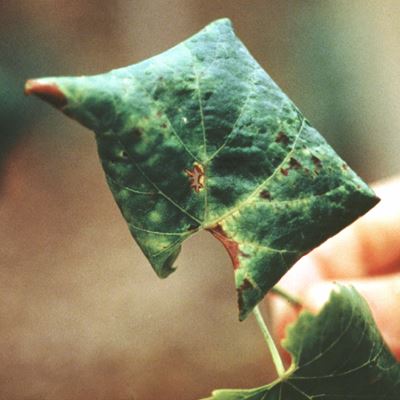This close-up photograph captures a fair-skinned person’s right hand holding a dark green, withered leaf between the thumb and forefinger. The leaf appears aged and damaged, with noticeable brown specks and browned edges, particularly where a piece has been chewed away by pests, revealing signs of blight. The leaf's veins are yellowish, and it has folded into a near-rectangular shape, akin to a small, shriveled pillow. Another green leaf is attached to it, which lacks the brown spots and has a green stem. The background is a blurry mix of greens, tans, and browns, suggesting a dirt ground beneath. The hand holding the leaf is slightly blurred, emphasizing the detailed texture and imperfections of the leaf in focus.